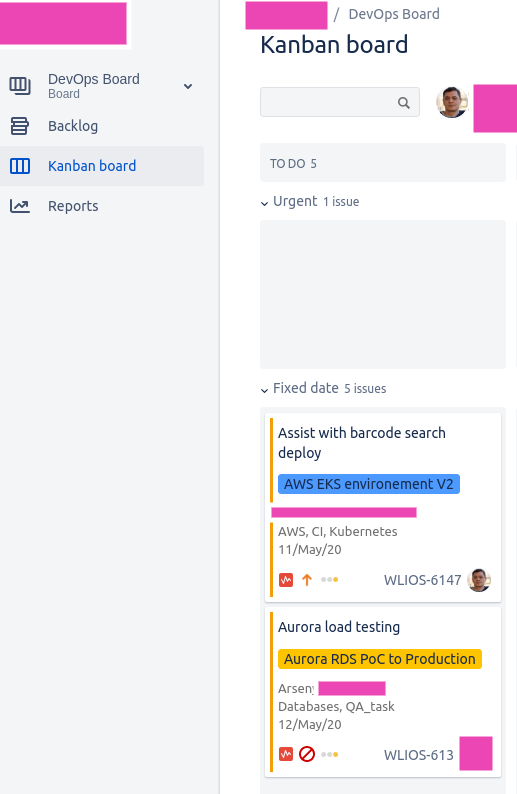This detailed description captures the layout and elements of a DevOps board with a split background. On the left, against a gray backdrop, various menu options are listed in black and blue text, topped by a hot pink rectangle labeled "DevOps Board" with a drop-down menu. The menu options include "Board," "Backlog," "Kanban Board," and "Reports." On the right, with a white background, a hot pink rectangle is placed in the top middle section, adjacent to black text stating "/ DevOps Board." Below, bold black text reads "Kanban Board," with a light gray search bar featuring a magnifying glass icon in the bottom right corner situated underneath. To the right of the search bar is an icon of a man with light brown skin, black hair, and brown eyes, wearing a gray shirt, followed by a hot pink square. Below these elements, a light gray rectangle labeled "To Do: 5" appears, accompanied by a drop-down menu mentioning "Urgent: 1 issue," followed by another light gray square. Further down, black text indicates "Fixed Date: 5 issues," also with a drop-down menu. "Assist with barcode search deploy" is written beneath this section. A blue rectangle follows, inscribed with "AWS EKS environment v2," leading to further details below it, such as "AWS CI Kubernetes 11 May 20" and "Aurora load testing."